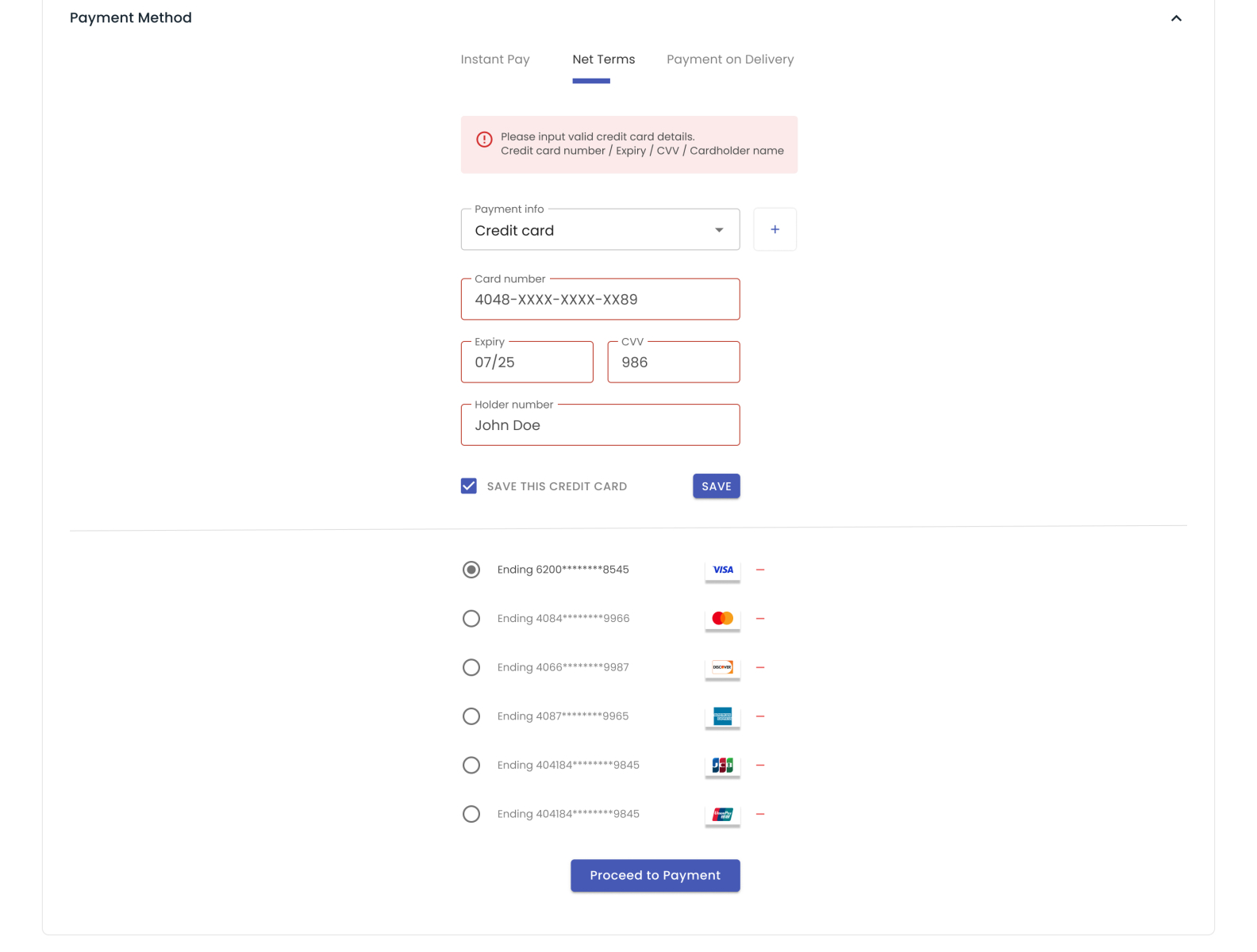The screenshot captures a section of a commerce website's payment page against an almost entirely white backdrop. In the top-left corner, the bold, black text reads "Payment Method." Centered on this page is a form for entering credit card details. The form fields, sequentially arranged, start with "Payment Info," defaulted to "Credit Card." The next field is labeled "Card Number," intended for entering the credit card number. Below this, two fields request the card's expiration date and CVV number, respectively. Following these, a field is designated for the "Cardholder Name."

Adjacent to a blue check mark for the "Save this card" option, there is a prominent blue button labeled "Save." At the bottom section of the screenshot, multiple previously stored payment methods are listed, each accompanied by a radio button to its left. The six saved cards display the type (Visa, MasterCard, etc.) and are partially obscured, showing only the beginning and ending digits of each card number for security purposes.